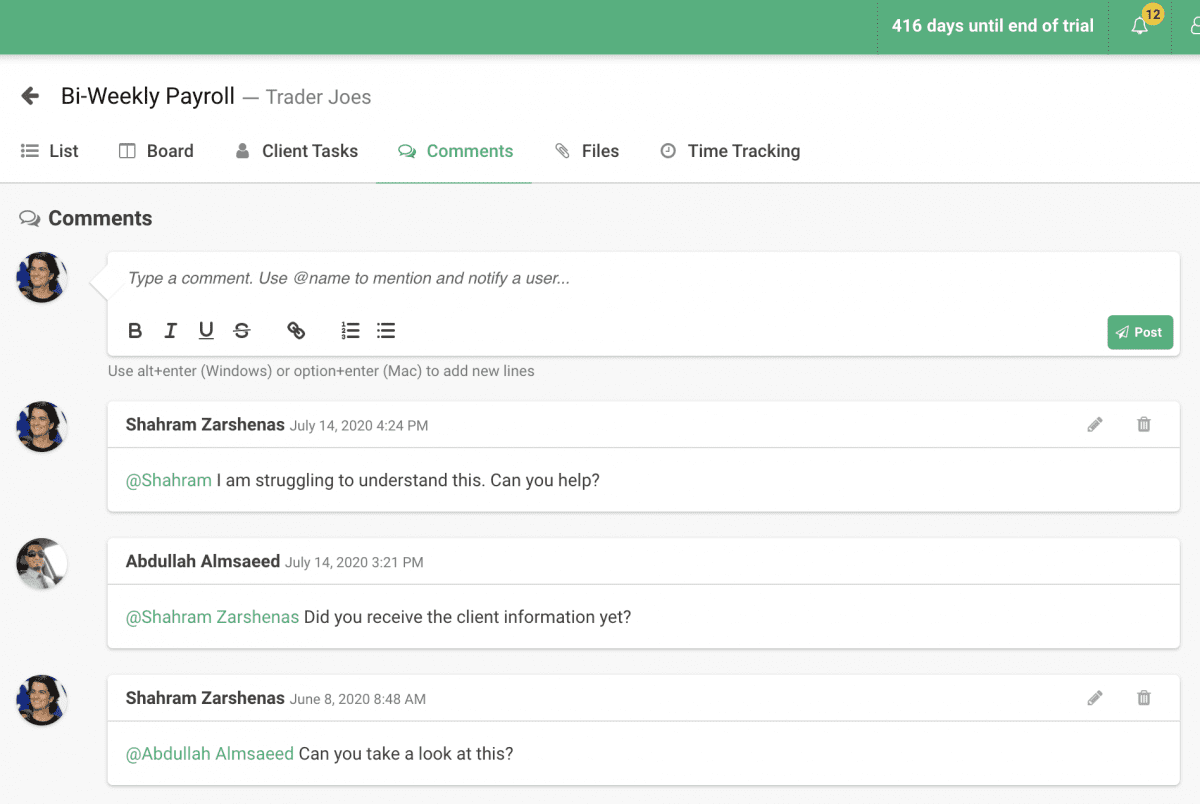Screenshot Description:

In the screenshot, a rectangular white background primarily dominates the screen of a computer or laptop. At the top of the page, there is a medium-colored green banner stretching horizontally from left to right. On the right side of this banner, a dark green vertical line separates a message written in white letters, "416 days until end of trial". Adjacent to this is a cluster of icons: a white bell icon next to a dark green vertical line, followed by a yellow circle with the numbers "12" in black, another dark green line, and a two-circle icon with a black arrow pointing left. 

To the right of this group, bold text reads "B-Weekly Payroll", and next to that, in light gray, the words “Trader Joe’s” with capitalized T and J. Following this section, there are three bullet points aligned with gray lines, accompanied by the word "List" beginning with a capital L. Beside this, an icon resembling a square containing a gray top line and a vertical middle line is visible. Further right, the word "Board" with a capital B appears next to the icon of a gray-colored person’s shoulders and head. Next to these, another set of words and icons include: "Client Task" with capital T, a green question mark icon beside the word "Comments" with a capital C, and finally, an icon resembling a paperclip next to the word “Files” with a capital F. Near this is a clock icon in gray, and the term “Time Tracking” with both T's capitalized.

Positioned below, a thin gray line runs horizontally across, separating the next section. This area has a light gray background with rounded profile pictures of individuals, starting with images of a woman. Below her image, gray lettering states, "Type a comment. Use @name to mention and notify a user..." followed by B-I-U icons, a strikethrough S, and several other formatting icons like bullet points.

On the far right, a green rectangular box with a dark green background contains a white triangle and the word "Post" in white lettering. Below this, in small light gray letters, it reads, “Use Alt + Enter (Windows) or Option + Enter (Mac) to add new lines”.

Further down, the image includes two separate gray-bordered text boxes with white backgrounds and black text. The first box shows a comment by "Sharam Zarshenas" dated July 14th, 2020, at 4:24 PM, followed by an at-mention in green text, "@Sharam", and a message in black text: "I am struggling to understand this. Can you help?" with a line separator beneath it.

Following this, another comment by a man wearing dark glasses and a shirt and tie is visible. His name, "Abdullah Almsied", in black text is timestamped July 14th, 2020, at 4:21 PM. The green text "@Sharam Zarshenas" precedes his message: "Did you receive the client information yet?”

Lastly, a response from Sharam Zarshenas, dated June 8th, 2020, at 8:48 AM, reads: "@Abdullah Almsied, can you take a look at this?" in black text. Each comment box has a pencil icon and a trash can icon to the right, along with gray line separators.